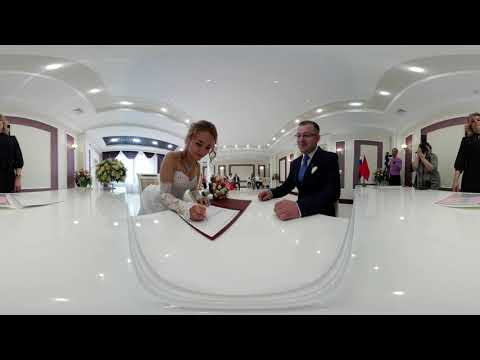In a pristinely white room illuminated by elegant lighting around the scalloped ceiling, a bride and groom sit at a large, marble-like white table. The bride, on the left, is in a wedding dress featuring intricate lace sleeves that reach mid-bicep. She holds a pen, poised over a document within a portfolio, which she is signing. The groom, on the right, is dressed sharply in a dark suit with a blue tie, black sports jacket, and a white pochette in his breast pocket. He has neat, short hair and wears glasses, attentively gazing at the document. The scene, formal and well-lit, is complemented by a background of other attendees, some seemingly capturing the moment with photography equipment. The entire setting exudes an air of ceremonial significance, possibly a marriage registration or similar event.